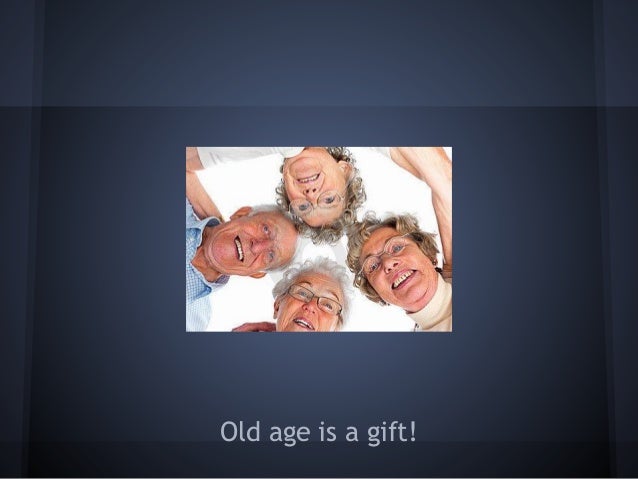In this image, we see what appears to be a PowerPoint presentation slide or possibly an inspirational advertisement. The background is primarily a dark gray color, with a lighter gray strip running horizontally across the top and a thin darker gray bar at the bottom, adding a contrasting touch to the design. On the left and right sides of the image, there's a slight gray beveled pillar effect, contributing to the overall aesthetic.

Centrally positioned is a ground perspective photograph of four elderly individuals, three women and one man, all smiling warmly as if they have just opened a gift and are peering down at the camera. The women, all with curly hair and glasses, are dressed in white shirts, while the man, who does not wear glasses, has white hair and is seen in a blue shirt. Their faces, which are tan, form a huddled circle and give a feeling of joy and camaraderie.

At the very bottom of the slide, in light blue text, is the message “Old age is a gift!” These words reinforce the theme of the image, emphasizing the positive aspects of aging and the joy of shared experiences.